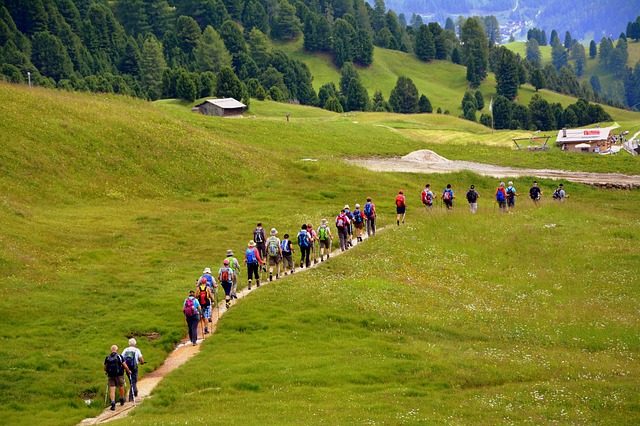The photograph depicts a group of more than twenty hikers, all equipped with backpacks and many using walking sticks, proceeding single file along a dirt path. The trail meanders through a verdant, open field with bright green grass dotted with small white flowers. The hikers, seen from behind and from a slightly elevated viewpoint, are dressed for warm weather in shorts and short-sleeved shirts. In the background, lush green hills rise, adorned with dense clusters of evergreen trees. On the distant left side, a barn is visible, while farther to the right, another building, possibly a house or workplace with an indistinct red sign, can be seen. The landscape is hilly, creating a picturesque countryside or rural scene with occasional patches of dirt and possibly a gravel area near the foreground.